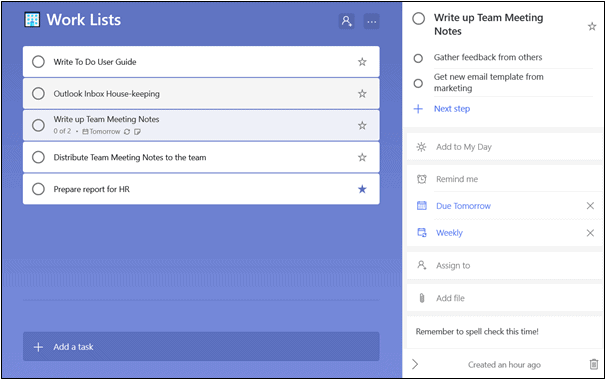The image displays a screenshot of a computer screen, prominently featuring a work task list application. The left two-thirds of the screen exhibit a purple-themed interface with the heading "Work List" at the top. Below the heading, there are six horizontally-aligned banners, each with clickable buttons and star icons for prioritizing tasks. The tasks listed on these banners are as follows:

1. "To Do List User Guide"
2. "Outlook Inbox Housekeeping"
3. "Wake Up Team Meeting Notes"
4. "Distribute Team Meeting Notes to the Team"
5. "Progress Report" (text is partially unreadable)

While the bottom task has been starred for priority, none of the tasks are checked as completed. A search magnifying glass icon is located at the top for easy navigation, and there is an option to add new tasks at the bottom.

On the right side of the screen, additional tasks and options are displayed:
- Task: "Write Up Team Meeting Notes"
- Task: "Gather Feedback from Others"
- Task: "Get a New Email Template for Marketing"

Highlighted prominently at the bottom right is a selected task: "Get Your Next Step." Accompanying tools to assist with task management include buttons for "Add to My Day," "Remind Me," and options to set due dates such as "Due Tomorrow" and "Weekly."

Overall, the application is designed to help the user organize their tasks effectively and ensure timely completion of work.